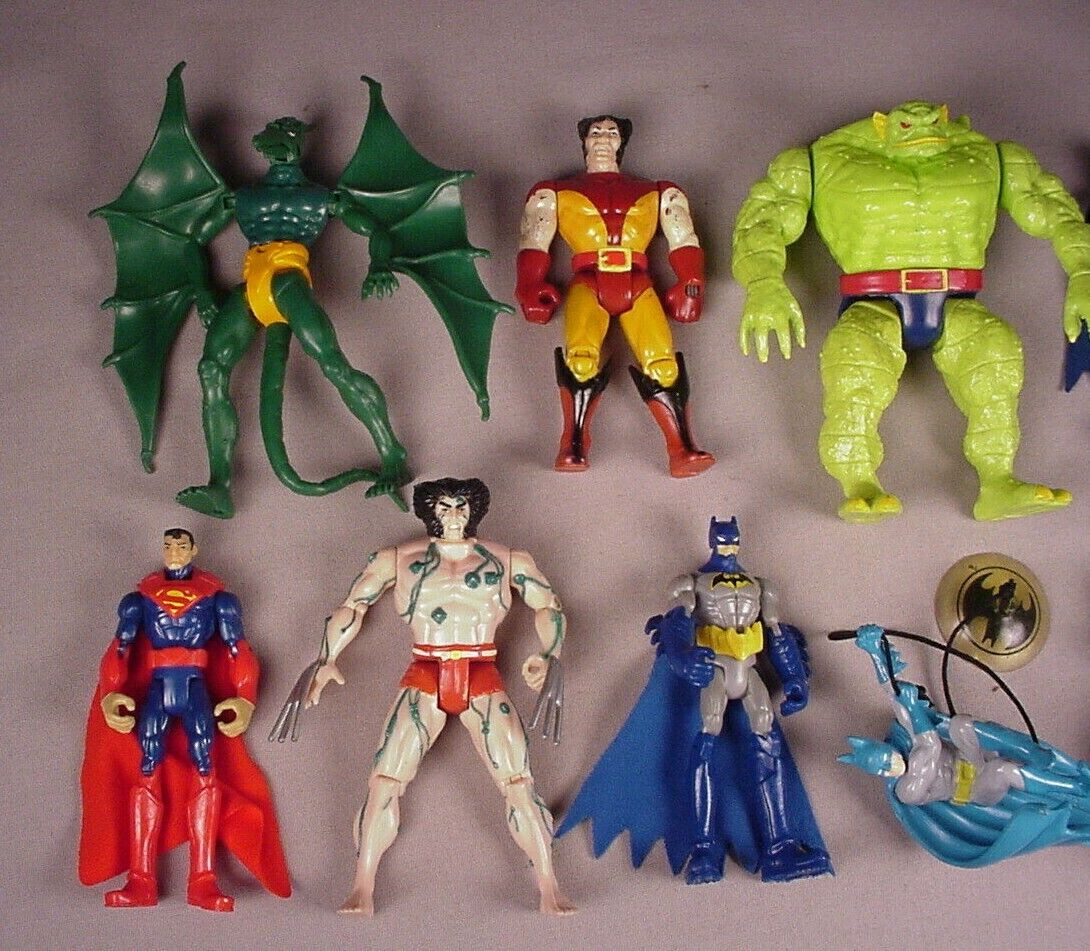This image showcases a collection of seven distinct action figures arranged on a grey backdrop. Prominently featured on the top left is a heavily muscled, dark green winged figure resembling a pterodactyl, identified as Sauron from Marvel Comics, adorned with a yellow belt and tail. To the right of Sauron stands an old-style Wolverine, recognizable by his brown and yellow costume. On the upper right side, there's a light green reptilian creature with human-like legs and blue-red attire. Towards the middle, you'll find a classic Superman donning his iconic red cape. Adjacent to Superman, there’s another formidable green character with a muscular build. At the bottom right side of the display, two Batman figures from DC Comics are noticeable; one showcases the character in traditional dark colors, while the other features a lighter colored variant. All these figures evoke a nostalgic sense of childhood and comic book culture.